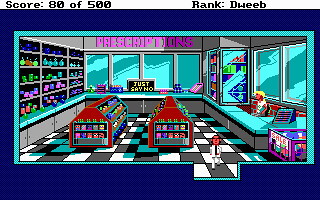This image is a screenshot from a retro computer game, likely from the 1980s, depicting the interior of a pharmacy. The scene is framed by a purple-blue border, with the top of the image displaying a score of 80 out of 500 and the rank "dweeb" in black text. The background showcases a black and white checkered floor, adding to the vintage aesthetic.

In the middle, the pharmacy is laid out with various shelves and counters. The left side of the store features brown shelves stocked with numerous bottles and packages, typical of a pharmacy. There are also two main aisles lined with triangular red shelves brimming with assorted items. The back wall hosts multiple windows, each allowing natural light to illuminate the interior. A prominent sign near these windows reads "just say no" in yellow letters.

On the right side, a person with blonde hair sits behind a turquoise counter, organizing goods. To their right, additional shelves hold more pharmacy products. At the very front right of the image, a sale bin marked "S-A-L-E" is visible. The rightmost section also includes two windows, and near the counter, additional items, possibly sweets or other small products, are displayed for purchase.

A character dressed in white, with black hair and a black tie, appears to be walking out of the shop, facing the viewer directly as though just completing their visit. The overall scene conveys the nostalgic allure and basic graphical style of early computer games.